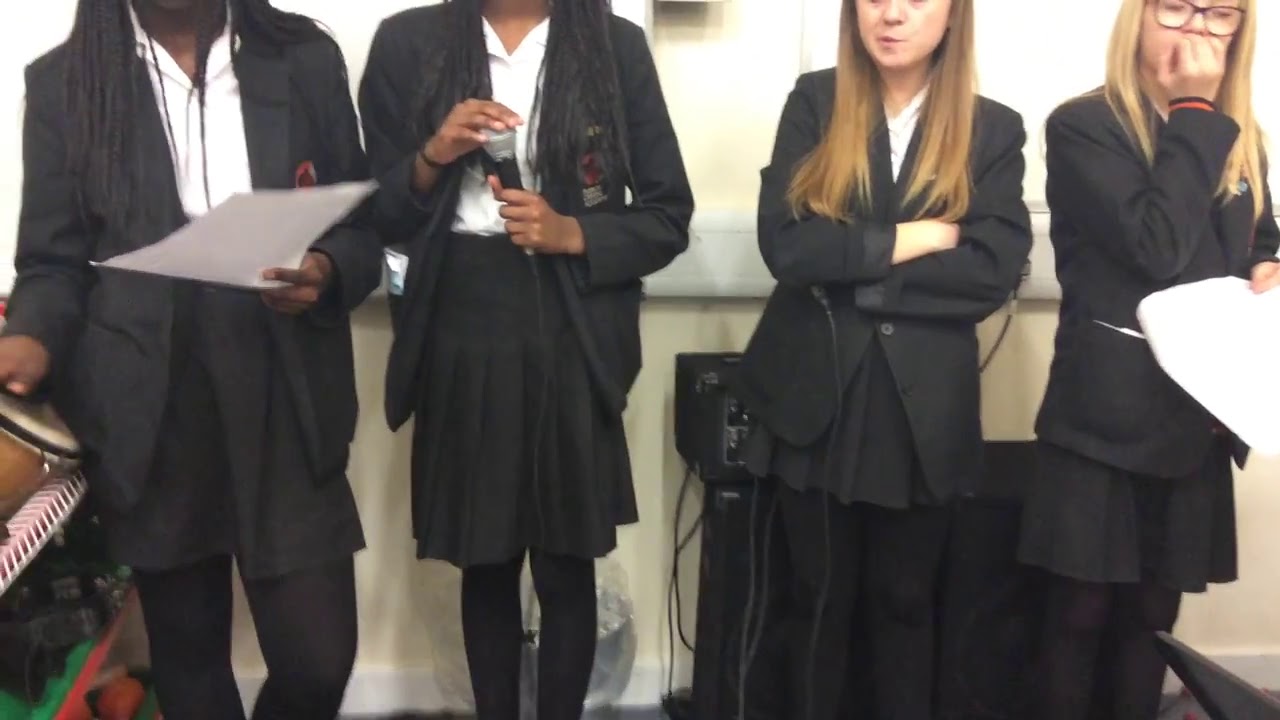The image captures four young individuals, seemingly three women and one man, standing side by side against a white backdrop, all dressed in matching business-like outfits. The attire consists of dark gray jackets, white blouses, black skirts for the women, and black tights or nylons; the man, depicted in a similar jacket, is wearing pants. The two individuals on the left, presumably African-American and whose heads are partially out of the frame, include one person holding a bongo drum with their right hand and another holding a microphone, partly concealed by their hand. In contrast, the two individuals on the right, likely Caucasian, include a woman with black-framed glasses, seemingly chewing her fingernails while holding a piece of paper, and another woman standing with her arms crossed and displaying a bored expression. The backdrop features some sound equipment, suggestive of a performance setting, thus hinting that these individuals may be part of a singing group.